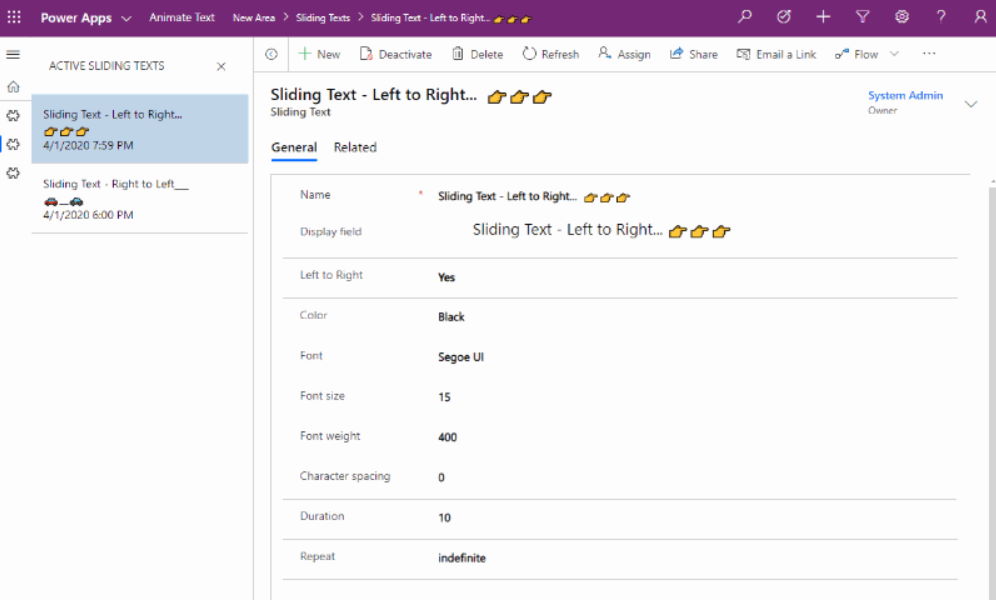The screenshot displays an interface dominated by a purple header at the top. Below the header are three rows of three dots each. The top section features a dropdown menu labeled "Power App" which includes options such as "Animate Text," "New Area," "Sliding Text Left to Right," and "Active Sliding Text." 

Subsequent lines detail a setting for "Sliding Text Left to Right" with an icon of a finger pointing to the right. There are additional sliding text options, including "Sliding Text Right to Left," illustrated with an icon of two cars moving left. Below these options, there are timestamps: "4-1-2020" and "7:59 PM" at the top and "6:00 PM" at the bottom.

Towards the middle, the interface shows categories "General" and "Related," with "General" being highlighted by a blue line. Detailed settings under "General" include configurations for "Sliding Text Left to Right," marked by three fingers pointing to the right. Specific parameters for the sliding text are noted, such as:
- Name: "Sliding Text Left to Right"
- Display Field: "Sliding Text Left to Right"
- Left to Right: "Yes"
- Color: "Black"
- Font: "Sugo-UT"
- Font Size: "15"
- Font Weight: "400"
- Character Spacing: "0"
- Duration: "10"
- Repeat: "Indefinite"

On the right side of the interface, the text "System Administration" is highlighted in blue with "Owner" listed underneath.